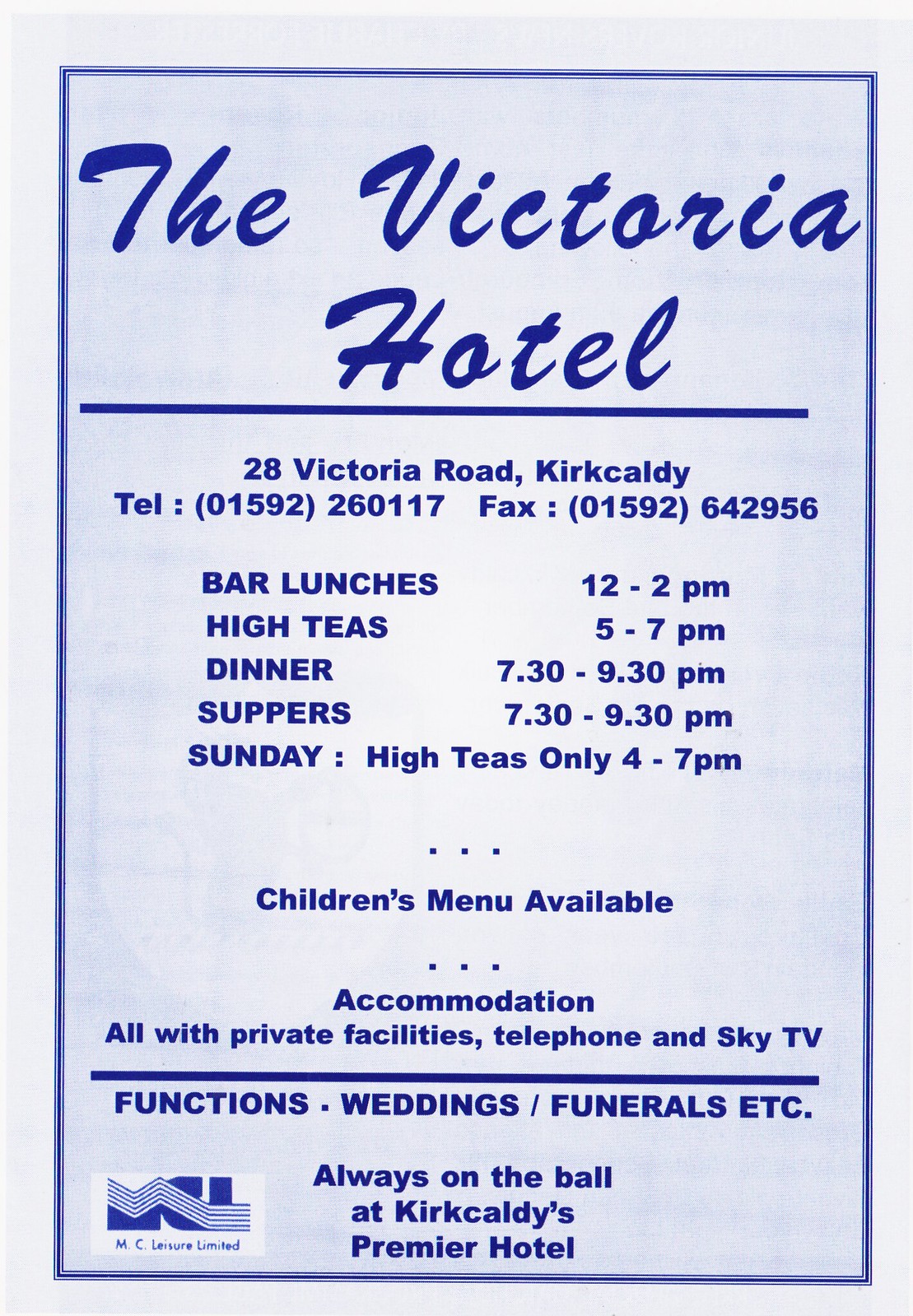This image is a print advertisement for the Victoria Hotel, likely designed for a magazine or newspaper. The ad features a gray border surrounding a light blue, rectangular text box in portrait orientation. At the top, in bold decorative cursive, "The Victoria Hotel" is prominently displayed. Below this, separated by a divider line, is the detailed contact information: "28 Victoria Road, Kirkcaldy, telephone 01592-260-117, fax 01592-642-956." The ad lists various services available at the hotel, including bar lunches from 12-2pm, high teas from 5-7pm, dinner from 7.30-9.30pm, and suppers from 7.30-9.30pm. On Sundays, high teas are available only from 4-7pm. Additionally, it notes that a children's menu is available. The accommodations offer private facilities, telephone, and Sky TV. The hotel also hosts functions such as weddings and funerals. The tagline "Always on the ball at Kirkcaldy's Premier Hotel" suggests a connection to sports, possibly soccer. Finally, the bottom left corner features the logo of MC Leisure Limited, which includes the stylized letters "MCU" with a zig-zag design.